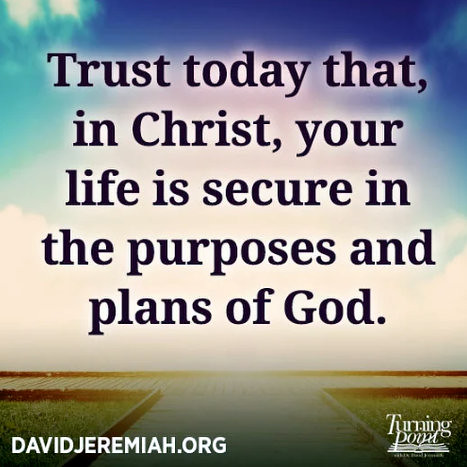In this graphic image featuring a quote likely derived from the Bible, the central element is a message in bold navy blue lettering that reads, "Trust today that in Christ your life is secure in the purposes and plans of God." The backdrop showcases a serene sky with varied hues—dark blue at the upper right, transitioning to lighter blue and eventually white toward the bottom. Below the sky, there's a wooden boardwalk forming the shape of a T, stretching away from the viewer and then diverging into paths leading left and right. The foreground includes some grass flanking the boardwalk. In the lower left corner, the text "davidjeremiah.org" is displayed in white. Meanwhile, the lower right corner features the "Turning Point" logo, depicted with text and an image of an open book. The overall composition combines elements of nature and faith, underscoring the uplifting message.